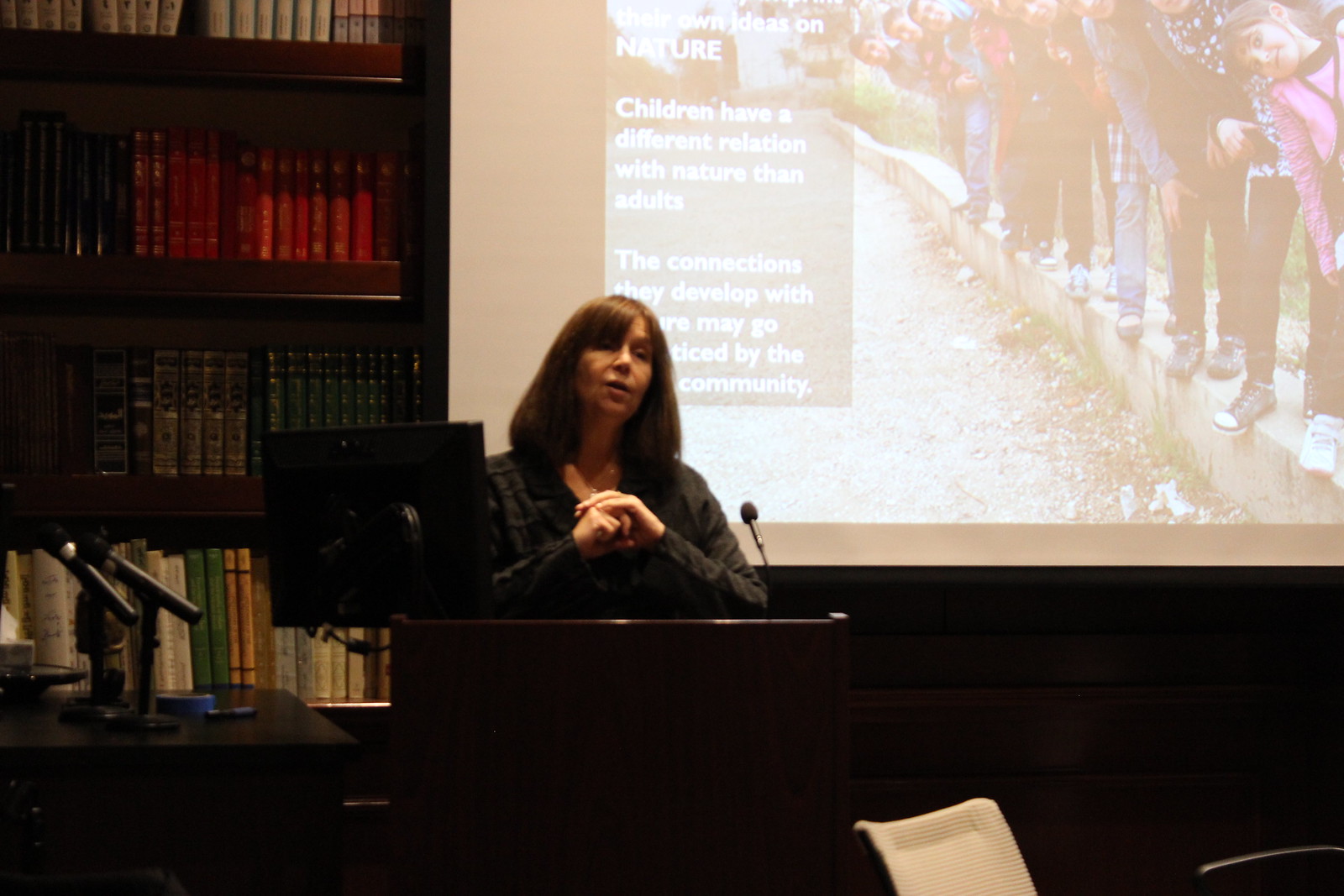This horizontal rectangular photograph captures a female presenter standing at a lectern with her elbows leaning on it, and a microphone positioned next to her left elbow. The woman, who has long hair, appears to be mid-speech, suggesting the photo could be a still from a video. Behind her, a faintly visible projector screen displays an image of children standing at the edge of something, with white text that discusses children's unique connection with nature. To her left, there's a tall bookcase filled with assorted colored books, indicating a potential library or old educational building setting with dark stained wood walls. The room is dimly lit, with the possibility of additional microphones or another lectern visible in the shadows, and a chair partially in view.